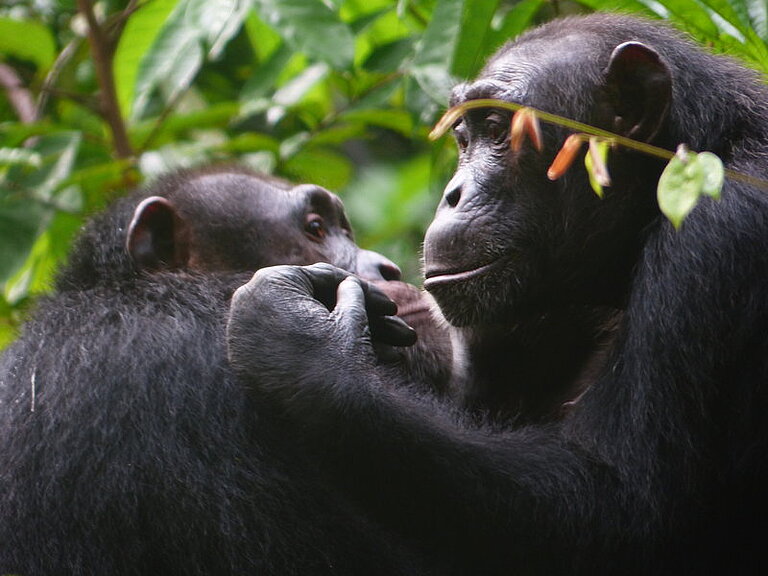The image features an intimate close-up of two black chimpanzees amidst a backdrop of lush green foliage. The chimpanzees are facing each other, with the older chimp on the left having smoother skin on its nearly bald head and a more prominent face, sitting in a low position. The larger, younger chimpanzee on the right is perched slightly above, resting its left arm gently on the older chimp's shoulder. Their faces exhibit a natural smile and curious eyes, directed off into the distance, suggesting something intriguing behind the photographer. Both chimps have thick hair covering their bodies, except for their exposed, almost hairless fingers. The intense focus on the primates creates a blurred background effect, where dark foliage dips down behind them. A vine with reddish and green leaves, bearing orange flowers, partially obscures the face of the younger chimp and adds a splash of color to the serene moment captured. They occupy about 80-90% of the image, underscoring their close bond and detailed expressions.